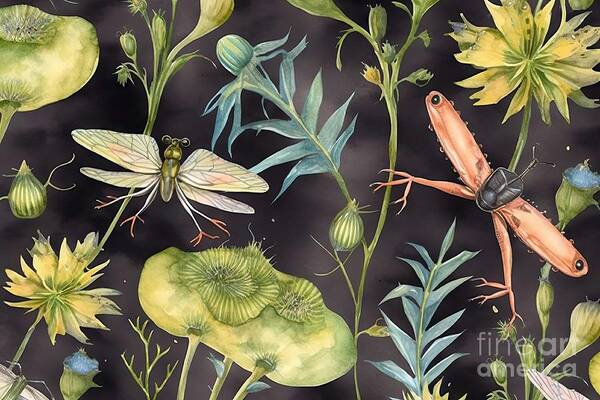This detailed painting, set against a dark black background, showcases a vivid collection of green and blue-hued plants and various insects. At the top left, a wire-like leaf extends into the scene, accompanied by a yellow plant with distinctive leaves. Nearby, at the top right, an insect with butterfly-like wings catches the eye, while a moth can also be seen fluttering within the composition. 

In the bottom right corner is a discreet, transparent watermark stating "Fine Art America." Surrounding it, there are several intriguing elements: a half-butterfly, half-insect creature, wings and leaves with visible veins, and a large beetle with its wings outstretched. Also present are a few yet-to-bloom flower buds. The combination of these plants and creatures, particularly dragonflies and moths, creates a striking nature scene where the elements seem to almost glow against the dark backdrop.